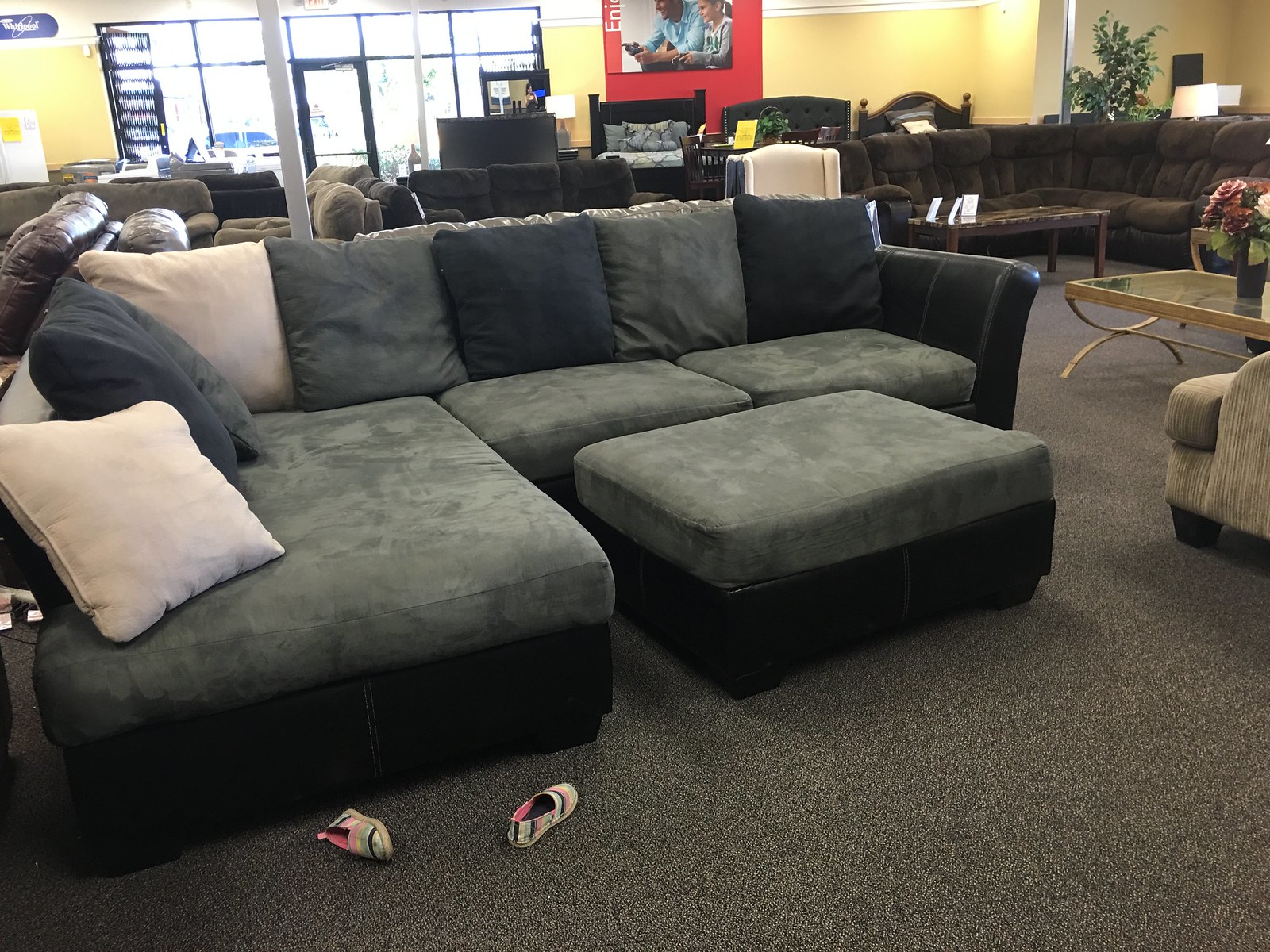The image depicts a bustling furniture store showroom with a variety of sofas and other furnishings neatly arranged on a dark-colored carpet. Dominating the foreground is a dark green L-shaped couch with black trim, adorned with an eclectic mix of blue, gray, and cream cushions. A pair of children's shoes, multicolored in hues of black, green, pink, and yellow, are casually placed in front of this couch, adding a touch of lived-in realism to the scene.

The background reveals an assortment of additional furniture, including a large brown L-shaped sofa paired with a couple of tables, emphasizing the store's extensive inventory. Visible through the multi-paned glass door and on the yellow walls are various signs, including a red one featuring an image of two people sitting, and a "Whirlpool" sign hinting at a possible appliance section. Beds with frames, coffee tables, and lampshades further diversify the space, with the shop's front windows casting ample light into the inviting, well-organized showroom. 

This detailed tableau creates a vivid picture of a well-stocked furniture and appliance store, highlighting the variety and arrangement of its offerings.